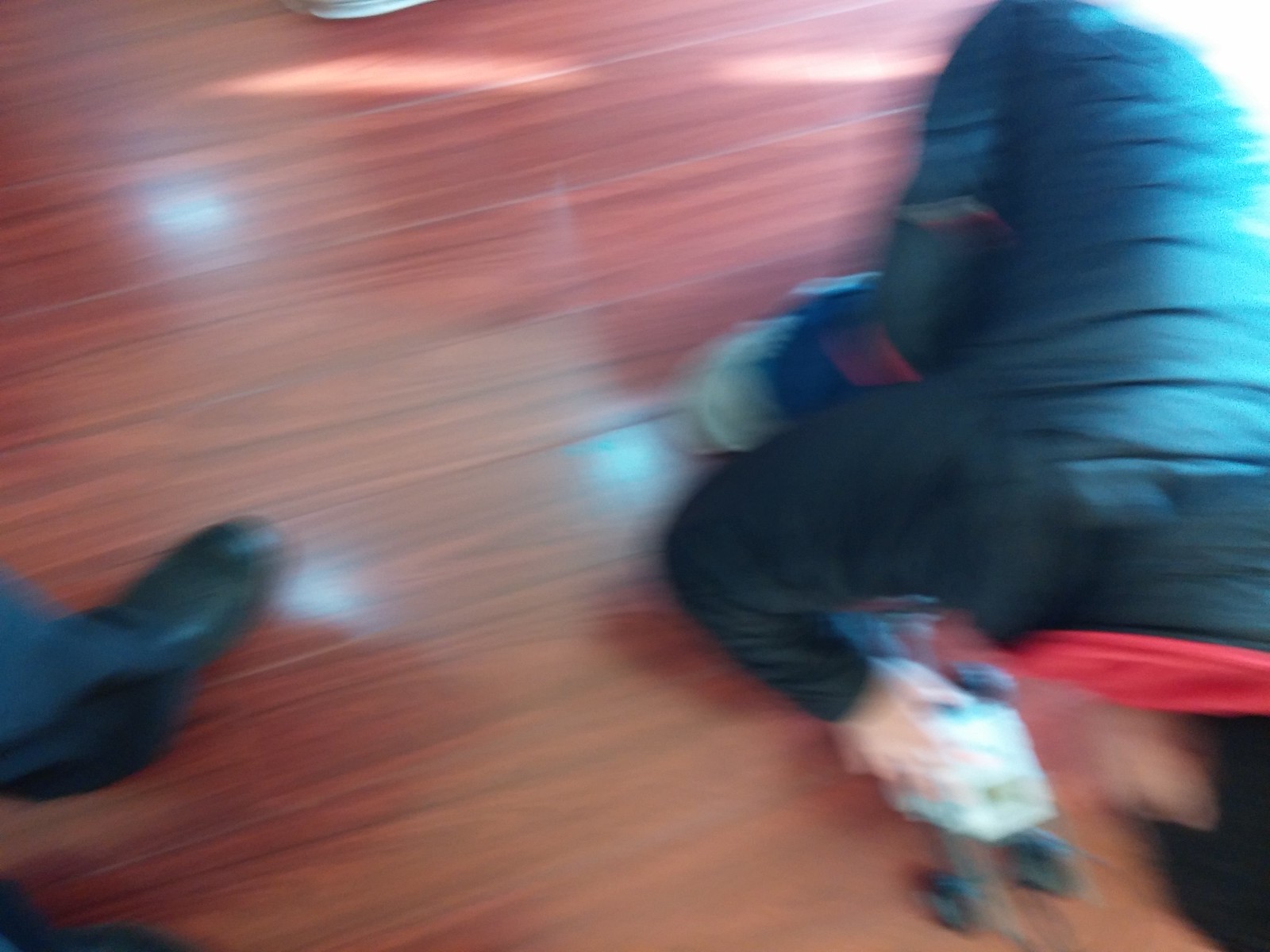A blurry photograph shows a partially visible person on a cherry wood floor. On the bottom left, a leg wearing navy blue pants and a black shoe is noticeable. The right side features the unclear outline of what appears to be someone's head in the lower corner, possibly holding an indistinct object. The individual seems to be wearing a winter jacket and could be crouching down, though the blur makes it difficult to discern their exact actions or direction they are facing.